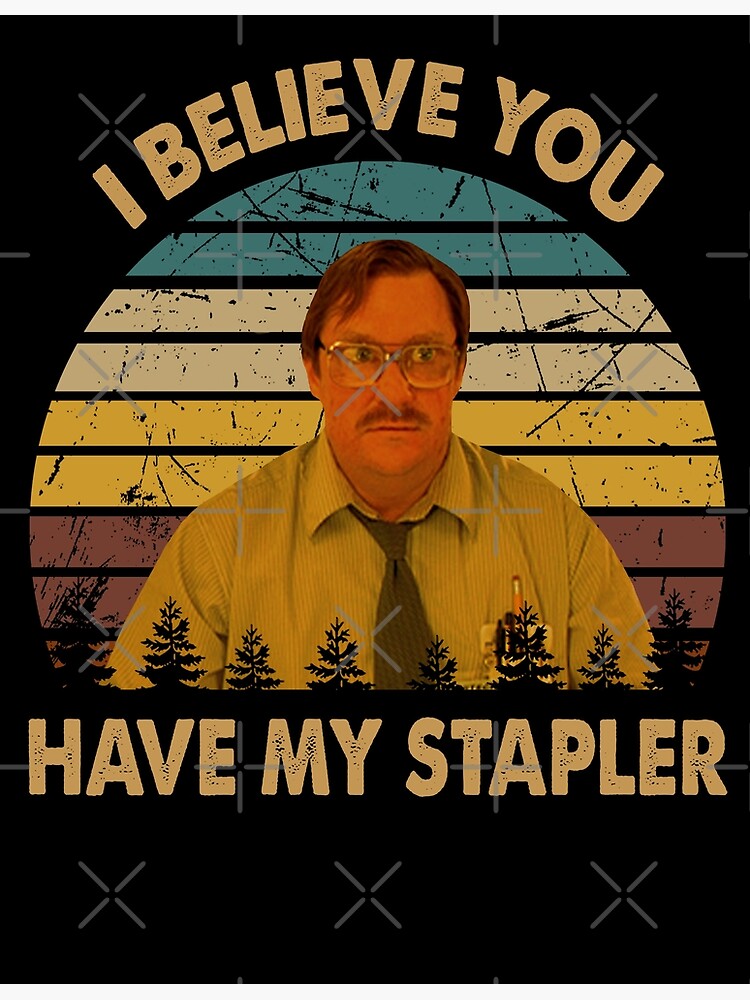The image features a white male character from the movie "Office Space," reminiscent of Dilbert, known for his awkward and disgruntled demeanor after being unknowingly fired. He is heavyset with a mustache, brown hair combed to the side, and thick, bottle-cap eyeglasses. He's wearing a green button-down collared shirt with a green tie, slightly loosened at the collar, and a pocket protector with a pencil sticking out on his left side. The background contains a bold, multicolored striped pattern with horizontal bands in blue, white, yellow, and purple, as well as black silhouette images of pine trees at the bottom. Above his head, in yellow capital letters, it reads, "I believe you," and below him, "have my stapler," referencing his catchphrases from the film. The entire scene is set against a black backdrop adorned with a pattern of plus signs and X's, partially cut off at the borders, potentially to prevent copyright infringement. The character's expression is one of confusion or anger, adding to the humorous and meme-like quality of the image.